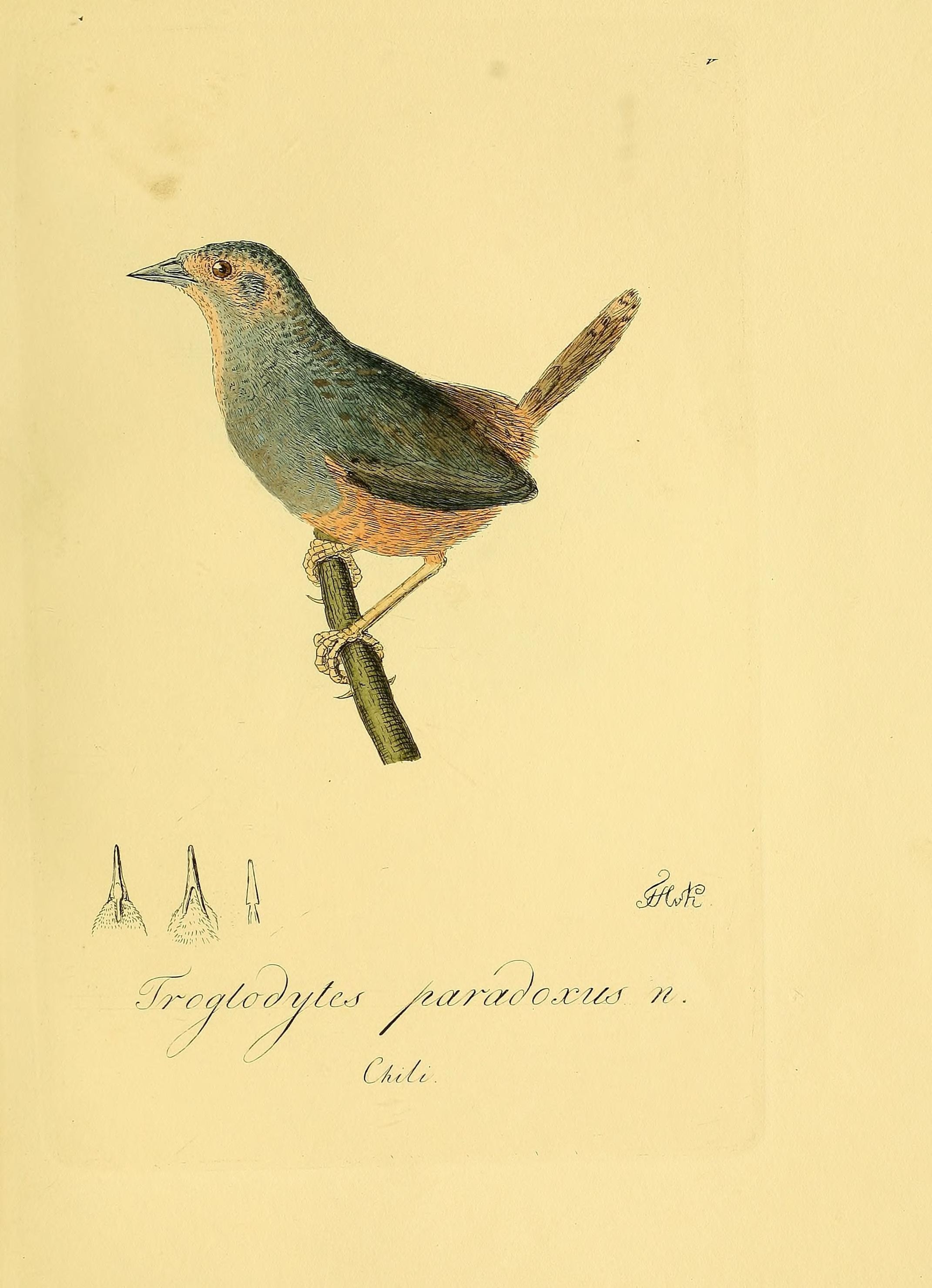The image depicts a detailed illustration of a bird perched on a thorny vine against a tan-beige background, reminiscent of an old 1800s taxonomy book. The bird is facing left, with its tail pointing towards the top right corner. It has dark green and yellow feathers with a bluish-gray breast, a gray beak, a striking dark brown eye, and yellow legs. The tail is golden-colored and quite prominent. The background suggests age with subtle smudges and an antique feel. Below the bird, in elegant cursive script, is the title "Troglodytes paradoxus" alongside some close-up renderings of beaks, suggesting a detailed study. Additionally, the artist's signature is in the lower right corner, further adding to its authenticity and historical allure.